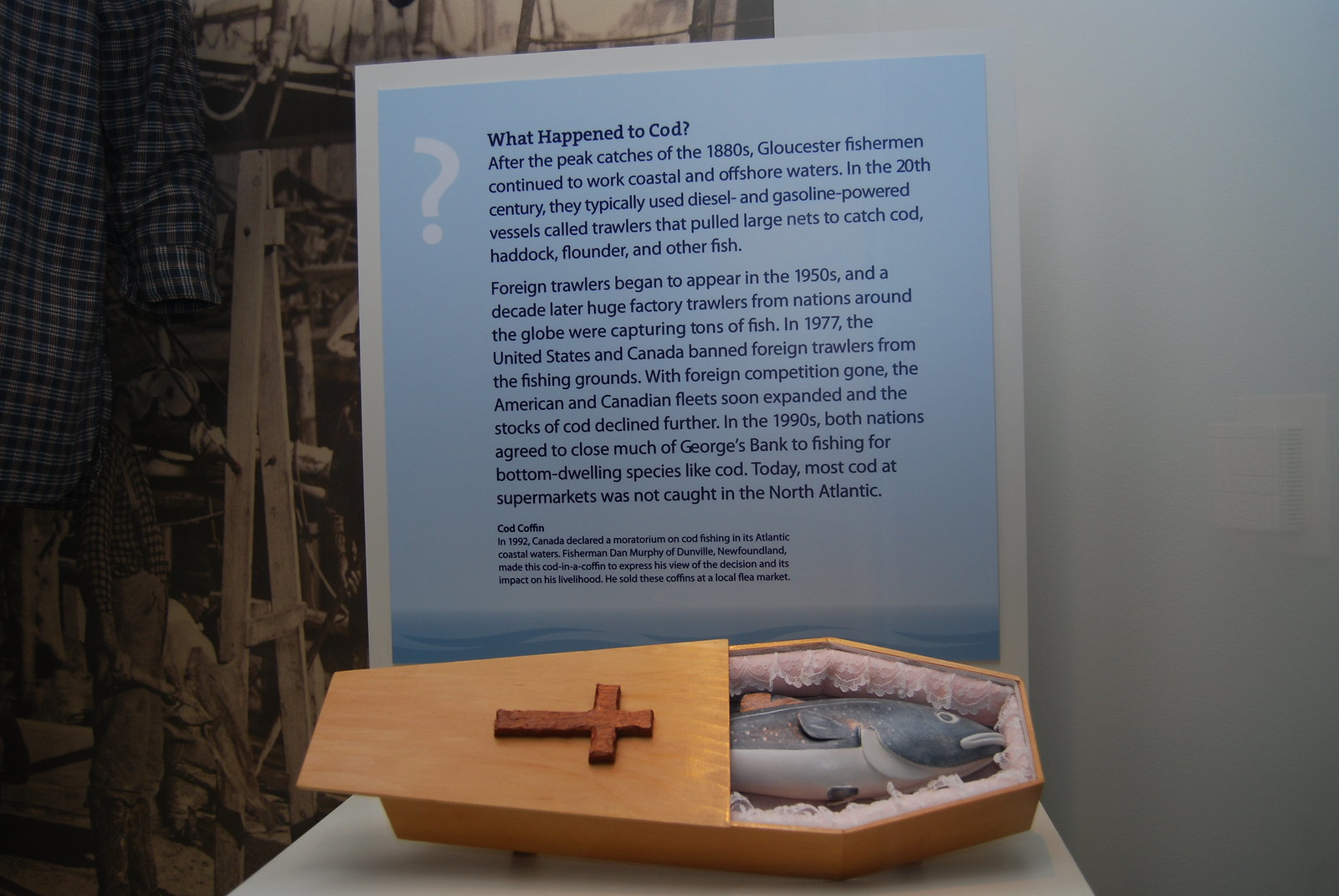The image in question is a detailed museum exhibit dedicated to the history and decline of cod fishing. At the center of the display is a light brown wooden casket, propped on a white square tabletop. The casket, which bears a prominent cross on its front, is partially open to reveal a gray cod fish lying inside, its eyes open and facing to the right. 

Behind this striking centerpiece is an informative display board with a light blue background and dark blue text titled "What happened to cod?" The text explains the historical context, detailing the peak catches of the 1880s by Gloucester fishermen, the transition to diesel and gasoline-powered trawlers in the 20th century, and the impact of foreign factory trawlers in the mid-20th century. It also covers the 1977 ban on foreign trawlers by the United States and Canada, and the subsequent measures in the 1990s to close off parts of George’s Bank to preserve cod stocks, noting the decline of North Atlantic cod availability in supermarkets.

To the right side of the background is an off-white wall, while to the left, a black and white photograph depicts fishermen working amidst what seems to be a tattered or industrial backdrop. Above this scene, a dark blue checkered shirt floats suspended in the air, adding a haunting, ghostly presence to the exhibit.

The display concludes with a footnote explaining the "COD coffin." This wooden casket with the fish inside was created by Fisherman Dan Murphy of Dunwill, Newfoundland, as a poignant protest against the 1992 Canadian moratorium on cod fishing, which critically impacted his livelihood. Murphy sold these symbolic coffins at a local flea market, underscoring the personal and economic distress caused by the moratorium.